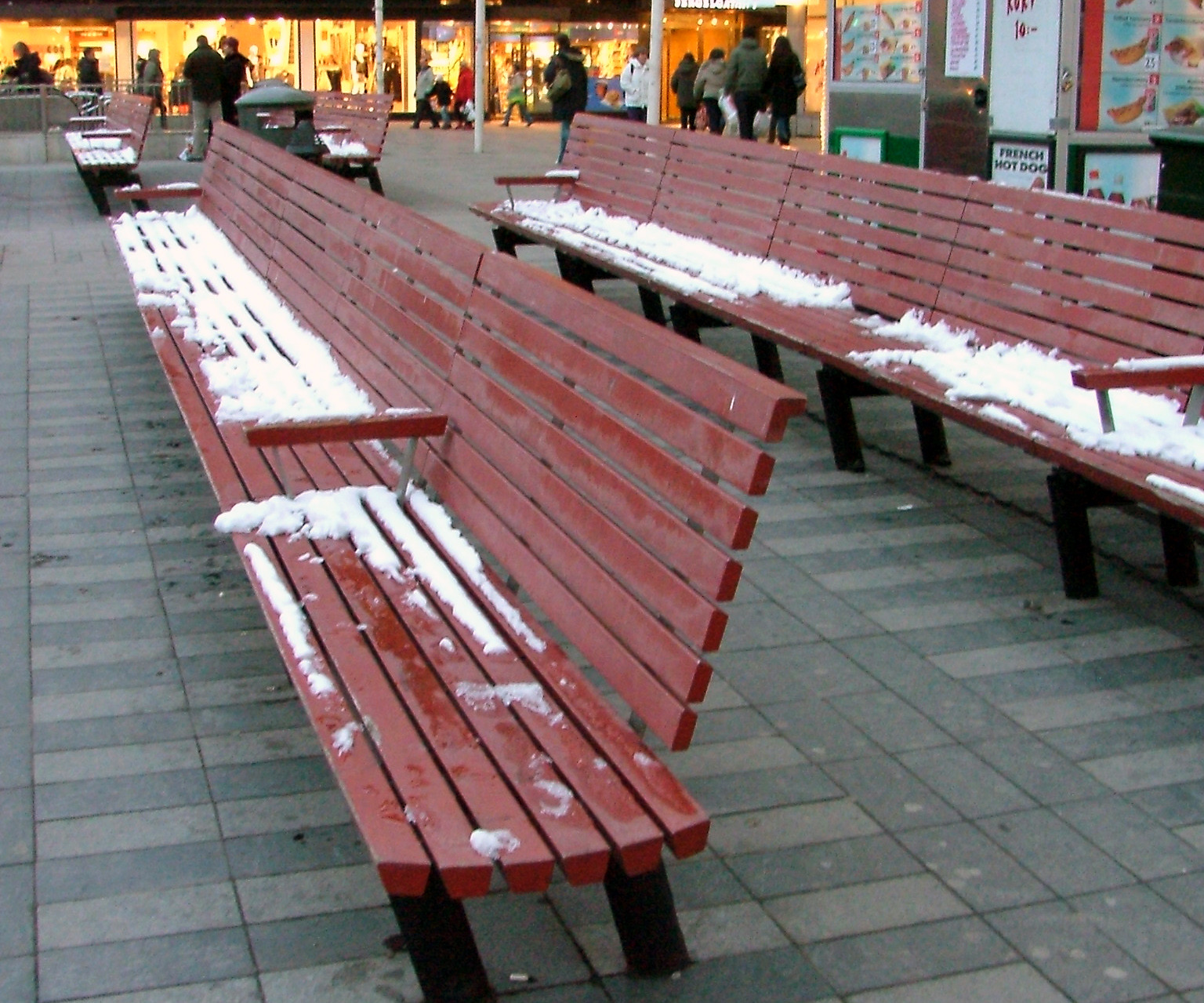The color photograph captures an outdoor mall or shopping center in winter. The foreground is dominated by several very long reddish-brown wooden benches, each around 15 to 20 feet in length, with random armrests. These benches have patches of snow on their seats, some wet spots indicating melting snow. The ground beneath the benches is tiled in grey, with varying shades. In the upper left and right corners of the image, illuminated storefronts can be seen, with some colorful signs on a wall to the right displaying what appears to be menus or advertisements, possibly for a restaurant offering items like French hot dogs. The background also features around a dozen people in heavy coats, walking and shopping. They appear as indistinct, shadowy figures due to the lighting. The atmosphere suggests cold weather, with no one seated on the benches.